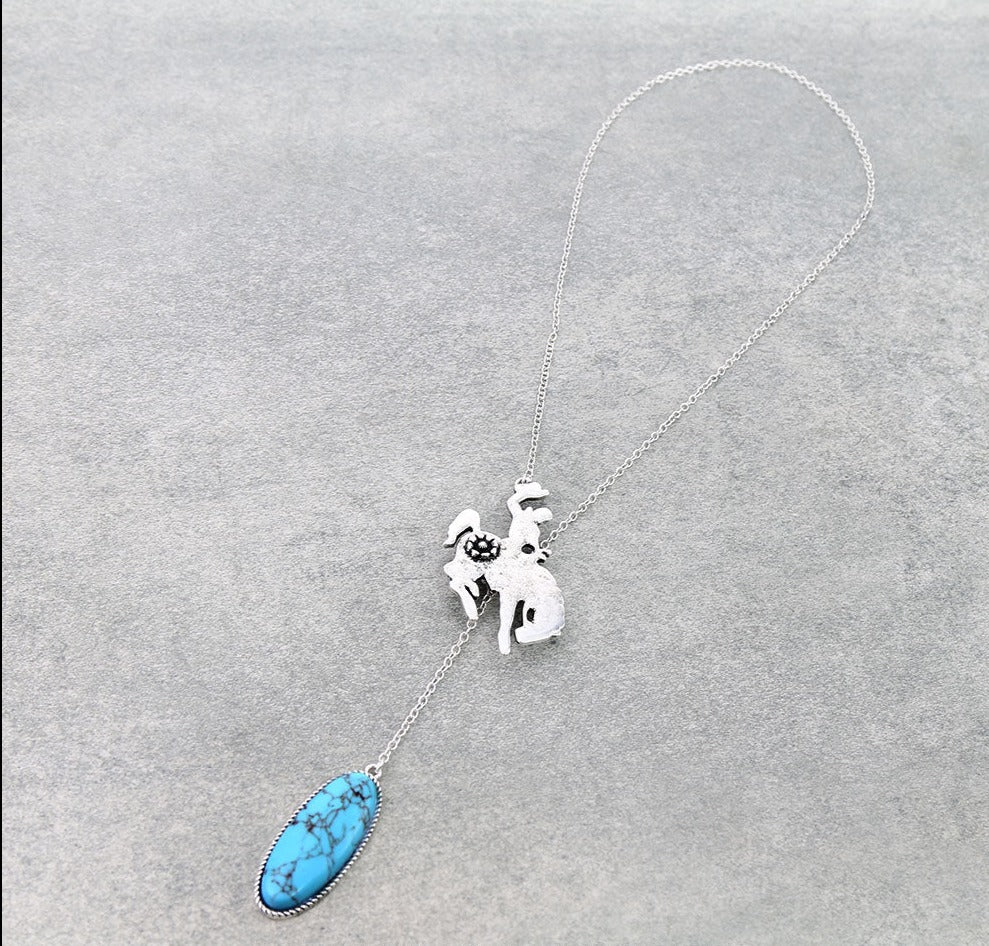This image showcases a silver necklace laid on a gray surface with a wide vertical rectangular frame. The necklace features a delicate, thin, silver chain. One end of the chain is adorned with an intricately designed silver pendant, depicting a cowboy riding a bucking horse. The cowboy is animatedly waving his hat in the air with one hand while gripping the saddle with the other. The horse is captured in mid-buck, with its head down and back legs kicked up, portraying a dynamic rodeo scene. There is a small silver circle with a central dot located towards the horse's back end. The other end of the necklace is highlighted by an elegant silver oval housing a striking blue stone. The stone is characterized by dark blue lines dispersed across its surface, adding depth and contrast to the piece. The entire composition is set against a consistent gray background, providing a neutral backdrop that accentuates the details and craftsmanship of the necklace.